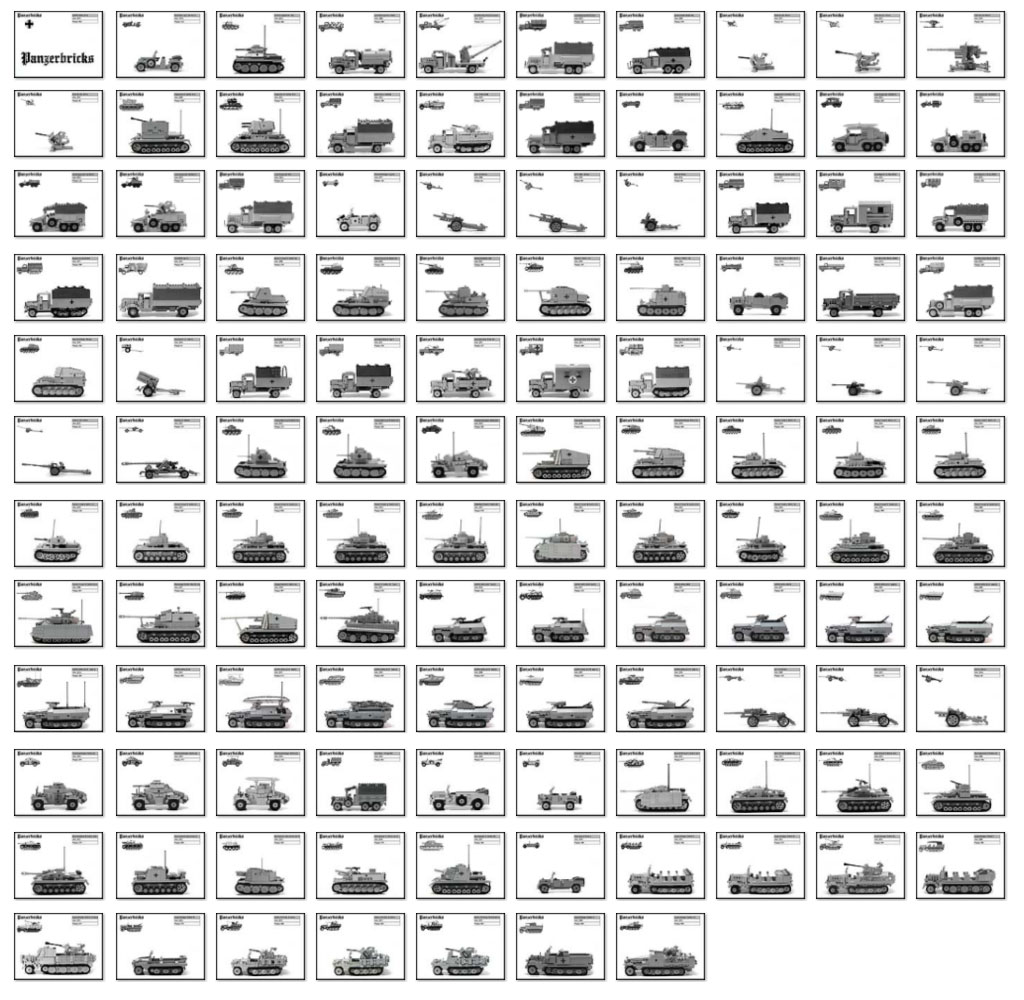The image displays a large, detailed chart featuring 117 small black and white illustrations of various military equipment arranged in a grid of 12 rows and 10 columns. Each box in the grid contains an image of a military vehicle or piece of artillery, accompanied by text at the top, though the writing is too small to decipher. The chart showcases a wide range of army armament, including tanks, trucks, towing vehicles, artillery pieces, engineering vehicles, small armored cars, self-propelled artillery, jeeps, half-tracks, and howitzers. The orderly array of the images suggests they might be representations of collectible toy models, possibly of German origin, given the mention of a German word in the first box.